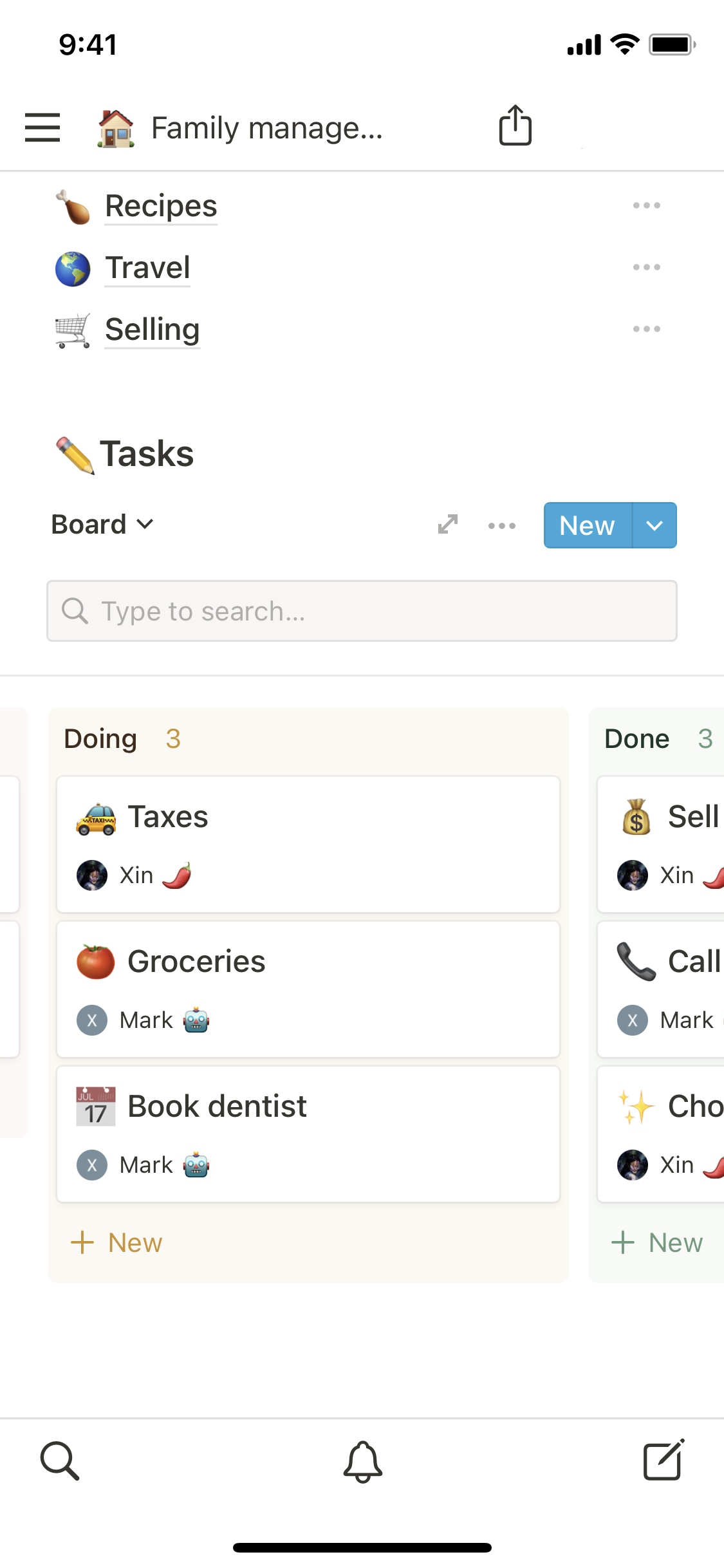The image is a detailed screenshot of a digital family management dashboard with various icons and labels. At the top, the status bar displays the time "9:41," with a Wi-Fi signal strength icon and a battery symbol. Below the status bar is a white background with black text. There are three horizontal black lines followed by a light tan and brown house icon, labeled "Family Manager." Next to this is a black box with a black arrow.

Descending further, there is a series of icons and labels:
- "Recipes" with a chicken drumstick icon.
- "Travel" with a green and blue globe icon.
- "Selling" with a silver shopping cart icon.
- "Task" with a yellow pencil icon.
- "Board" with an adjacent search box and a magnifying glass icon.

Above the search bar, there is a blue and white box labeled "New." Below the search bar, under the label "Doing (3)," are several white boxes:
- "Taxes" with a yellow car icon.
- A picture of a person labeled "Xin" with a red chili pepper icon.
- "Groceries" with a tomato icon.
- "Book Dentist," marked with a white and red calendar icon and the name "Mark," along with a blue robot icon.
- Another white box labeled "New" in gold.

On the partial right side of the image, there is text that is not fully visible but includes:
- "Done (3)"
- "Sell" with the name "Xin" and a chili pepper icon, alongside a tan money bag icon.
- "Call" with a grey phone icon and names "Mark" and "Cho," accompanied by gold stars.
- The name "Xin" appears again with a chili pepper icon and a "New" label.

At the bottom of the image are three icons: a magnifying glass, a bell with a black line underneath, and a box with a pencil.